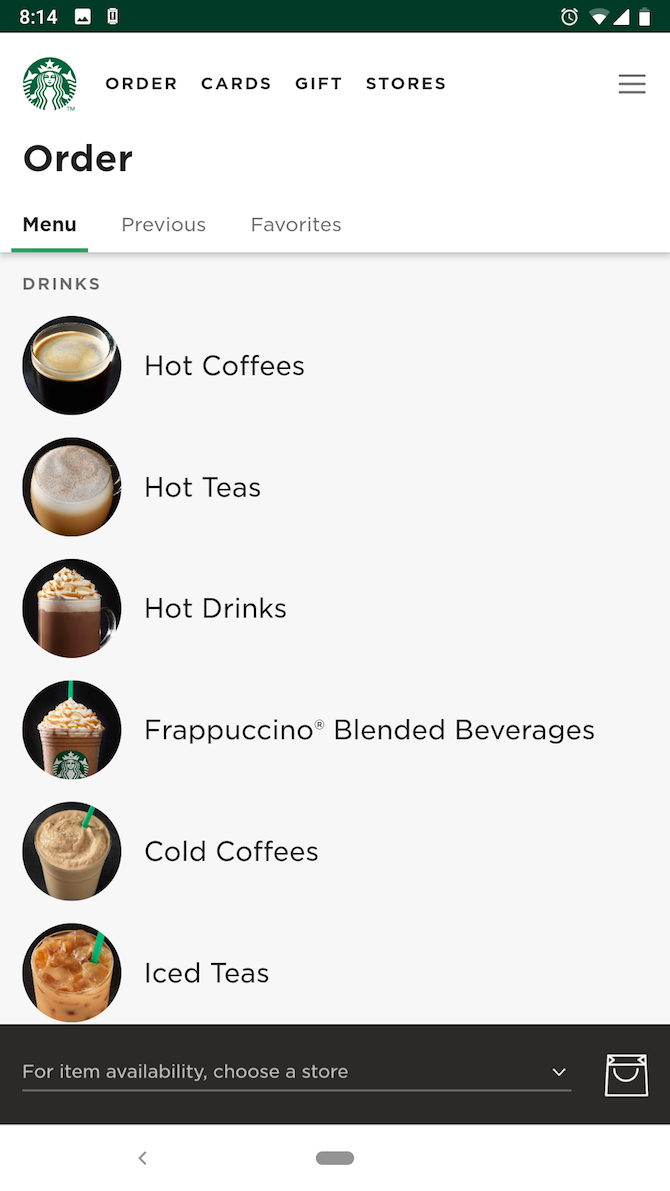The image depicts a smartphone screen displaying a Starbucks ordering menu. 

In the upper right-hand corner, a green bar with the time "8:14" is visible, alongside an alarm clock icon, Wi-Fi signal bars, and a battery icon. The Starbucks logo is prominently positioned in the upper left-hand corner.

Beneath the logo, navigation options labeled "Order," "Cards," "Gifts," and "Stores" are neatly aligned across the top. The word "Order" is prominently displayed below these options, indicating the current section of the app being viewed.

The menu is divided into three categories, with one highlighted by a smaller green line and another by a solid line, indicating the current selection. The options are "Menu," "Previous," and "Favorites." The "Menu" section is expanded to display various drink categories, including "Drinks," "Hot Coffees," "Hot Teas," "Hot Drinks," "Frappuccino Blended Beverages," "Cold Coffees," and "Iced Teas."

Each drink category is accompanied by an illustrative image: 
- A dark coffee for "Hot Coffees."
- A steaming cup for "Hot Teas."
- A beverage with whipped cream for "Hot Drinks."
- A classic Frappuccino for "Frappuccino Blended Beverages."
- A cold coffee for "Cold Coffees," and an iced coffee for "Iced Teas."

Three of these five images feature the iconic green Starbucks straws, adding a touch of brand recognition to the visuals.